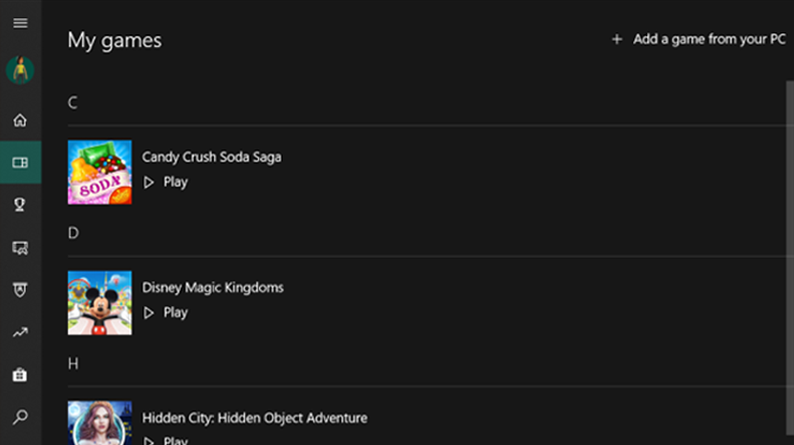The screenshot depicts a cropped view of the "My Games" section on a Windows PC, with dark mode enabled. At the top of the section, the heading "My Games" is prominently displayed. To the right of this title, there is a button labeled "Add a game from your PC." To the left of this button, an additional drop-down menu is visible. 

Beneath these elements, the user’s avatar is displayed on the left side. The avatar is a green icon featuring a person in a yellow shirt. Several navigation options are listed below the avatar, including "Home," "My Games," "My Rewards," "Accomplishments," and a Search button. At the moment, the user is navigating through their game library and is currently viewing the section for games that start with the letter "C."

The first game shown is "Candy Crush Soda Saga," which is represented by a thumbnail image and is accompanied by a play button. Immediately beneath this, the letter "D" is present, listing "Disney Magic Kingdom" with a Mickey Mouse thumbnail. Following is the letter "H" with the game "Hidden City: Object Adventure," depicted by a thumbnail of a lady and also featuring a play button. The person appears to be scrolling through their game collection on their PC.